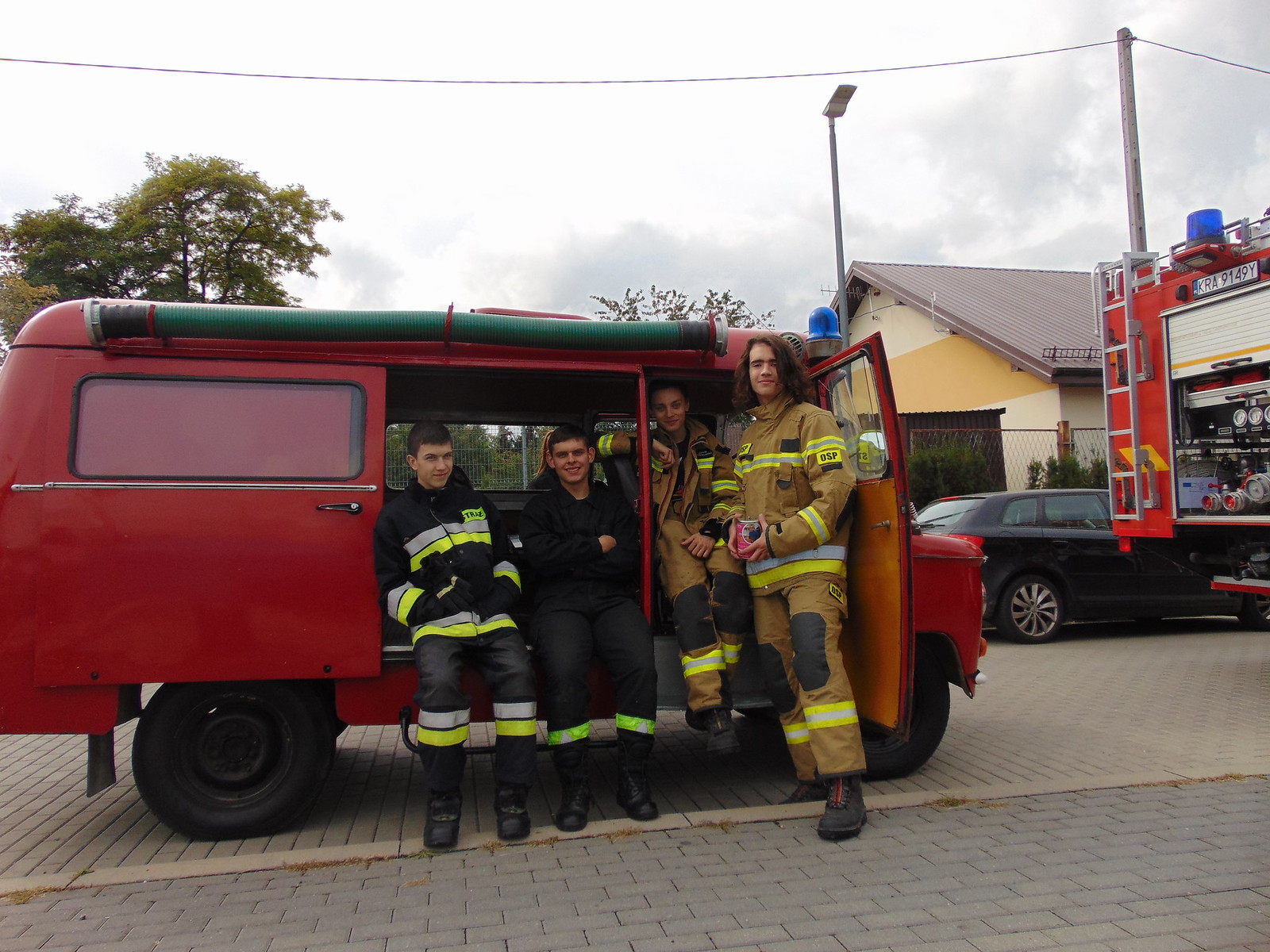This image features a detailed scene of four young individuals, three men and one woman, dressed as firefighters posing inside an old, classic red van, likely from the 1940s or 1950s. They are all smiling at the camera, donning full firefighter suits without helmets. The suits vary in color: two are wearing traditional brown suits with yellow and gray stripes, one on the far left is in an all-black and gray suit with light green reflective elements, and all of them have boots with reflective strips.

In the background, the overcast sky is white with gray clouds, featuring power lines and light poles. To the right of the van, there's a modern fire truck partially visible and a black car near it. A house with a yellow and off-white facade and a gray roof, along with a couple of trees, further frame the scene. The van, with its doors open, has black wheels and a green hose attachment, suggesting it is a parade vehicle showcasing vintage firefighting equipment. One of the individuals is holding a pink cup in both hands, adding a casual touch to this otherwise professional setup. The brick road beneath them emphasizes the quaint, historic feel of the scene.